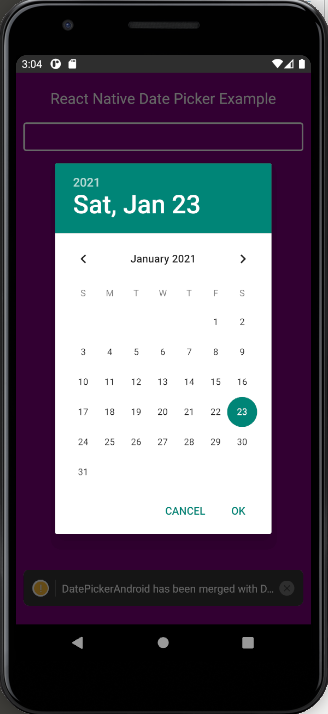Screenshot of a React Native Date Picker Example against a purple background. The date picker interface displays a calendar for January 2021, with "SAT" for Saturday and "JAN 23" highlighted with a blue circle. The left and right arrows allow for navigation between months. The days of the week are noted with "F" for Friday and "S" for Sunday, with the number "1" under Friday and "31" under Sunday. At the bottom, cancellation and confirmation buttons labeled "Cancel" and "Okay" are presented. Additionally, a notification indicates that "Date Picker Android has been merged with D..." Almost at the bottom of the screenshot, there's a black rectangle with icons in white, containing a left arrow, three dots, a circle, and a square.